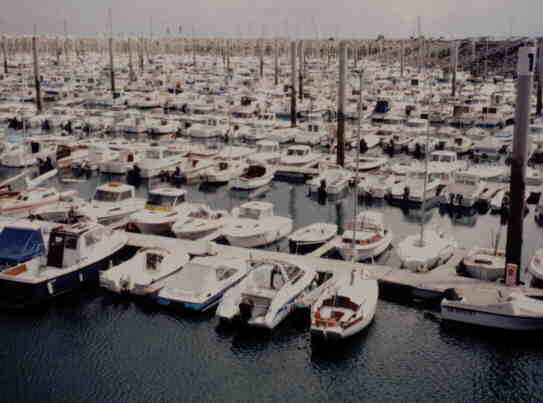This aerial view captures a sprawling marina with numerous wooden docks extending into a vast, flat, dark gray body of water, possibly a large lake or the ocean. The docks are lined with a multitude of boats, mostly small in size, parked side by side in a tightly packed manner. These boats come in various colors including blue, red, black, and the predominant white. Among the boats, there are sailboats with masts raised and a mix of rowboats and motorboats. Tall pilings are visible on some docks, likely to allow the decks to rise and fall with the water level. The scene has an aged appearance, giving it a vintage feel. In the background, a gray sky looms over what looks like the basin edge, enhancing the sense of an extensive, bustling harbor. With four prominent, double-sided piers and numerous passageways dividing the slips, it is estimated that there are several hundred boats depicted in this expansive and detailed marina setting.